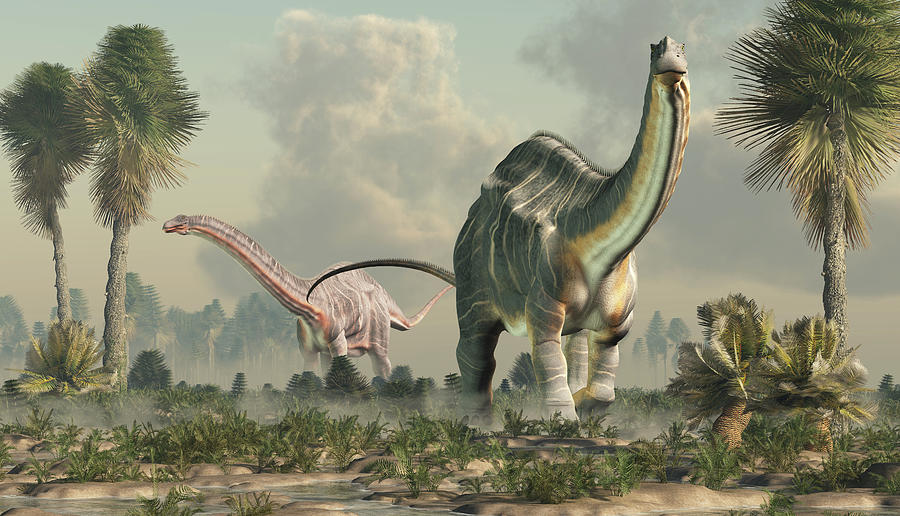This computer-generated illustration portrays a vivid prehistoric scene featuring two towering, long-necked dinosaurs in an open, tropical landscape. Dominating the foreground is a massive green dinosaur characterized by its four sturdy legs, elongated neck, curved back, lengthy tail, and a distinctive coloring pattern with beige stripes down its back and lighter green and yellow hues on the underside of its neck. Positioned further back is a similarly structured dinosaur, rendered in varying shades of reddish-brown with hints of gray and white. Surrounding these majestic creatures is a lush environment punctuated by tall, palm-like trees with slender trunks and green, stick-like leaves, as well as denser clusters of tropical plants and date-like trees near the bottom right corner. The ground beneath them is a mix of grass and brown dirt, all set against a backdrop of light blue-gray skies filled with fluffy white clouds and subtle, smoky shapes, enhancing the timeless atmosphere of this ancient landscape.